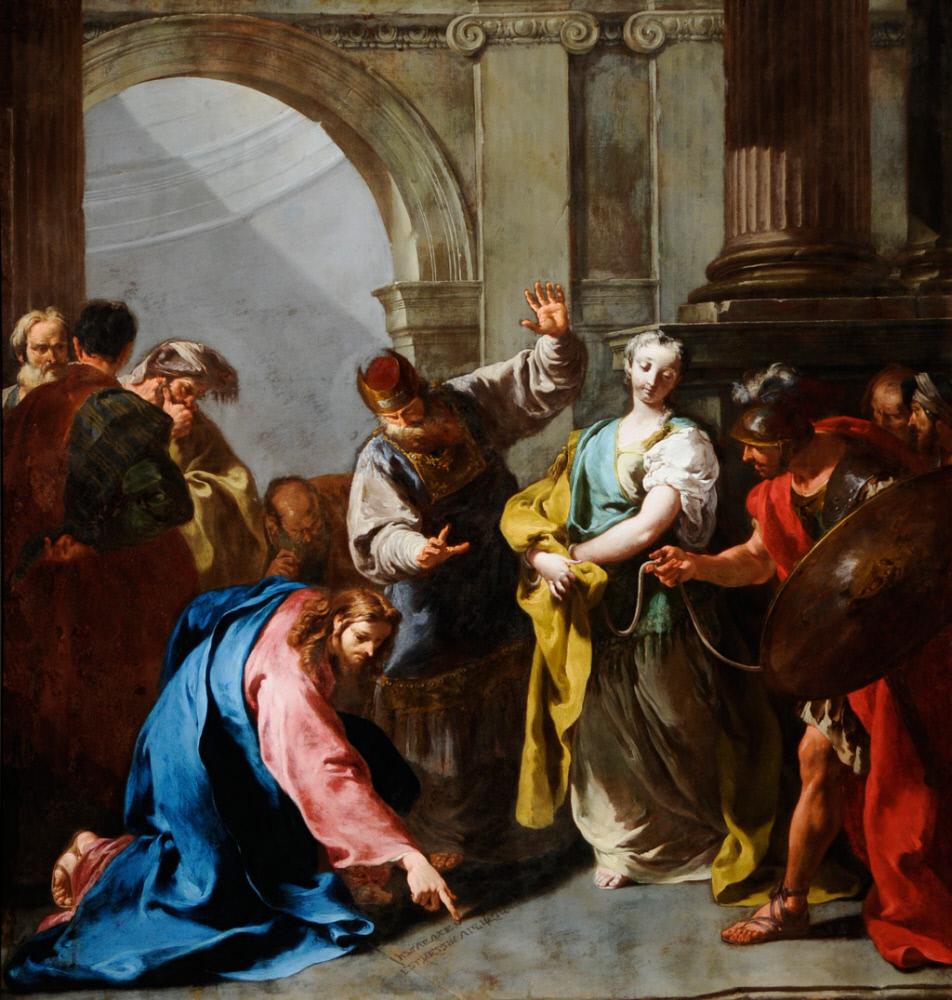In this detailed Renaissance-style oil painting, Jesus Christ, with his long brown hair and beard, kneels in the lower left corner, dressed in a light blue gown over a long-sleeved red or pink garment, pointing to inscribed sins on the stone floor. The scene depicts the biblical episode of a woman accused of adultery, who stands to the right, looking somewhat smug, with her wrists bound by a rope held by a Roman soldier gazing down at the writing. Flanking Jesus are astonished men, including a figure with a monocle in the far background, examining the script closely. The backdrop features grand stone columns and an archway, the right column appearing brown or bronze, with a light gray stone archway to the left. The painting is filled with vibrant colors, notably red, yellow, gold, blue, pink, white, beige, brown, and black, and is set in a vertical rectangle format. Surrounding figures include a bearded man in a red cap with his left hand raised in surprise, positioned center-right, others talking or peering intently at the ground, contributing to the dramatic ambiance of this religious masterpiece.